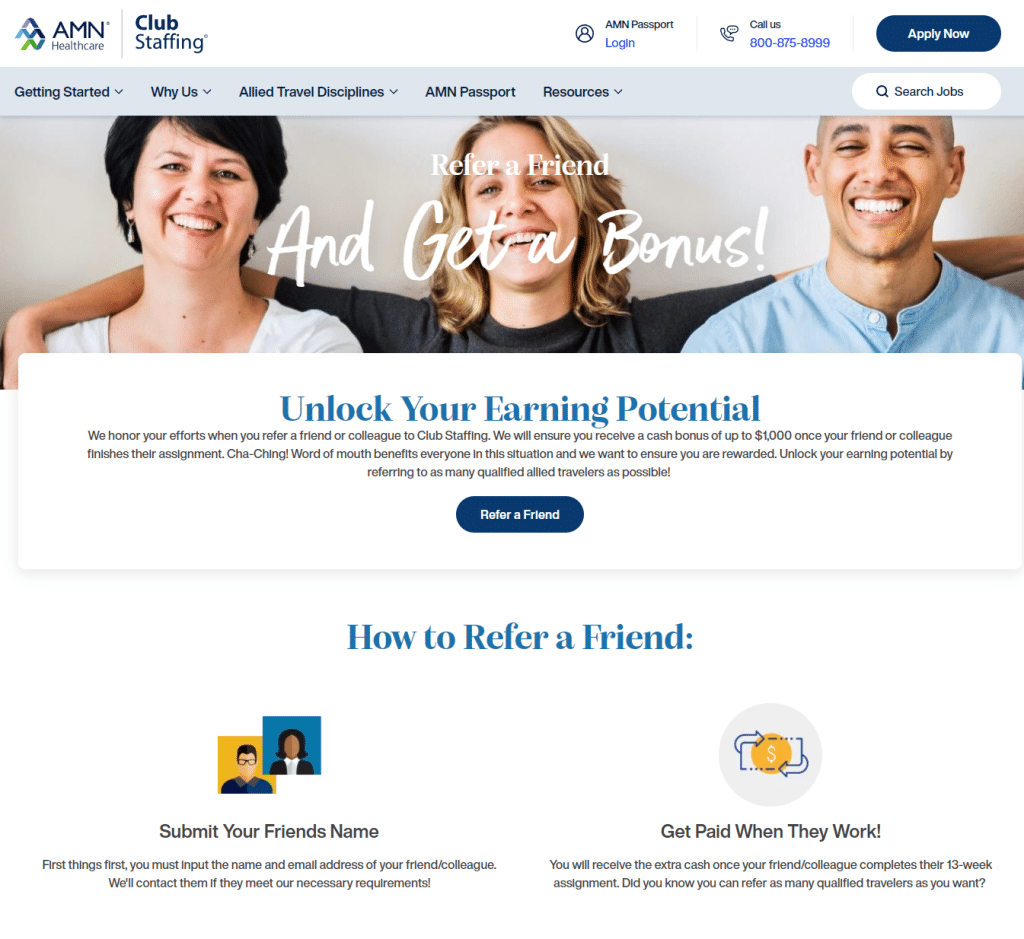This image is a screenshot from the AMN Healthcare website. In the upper left corner, the "AMN" logo is prominently displayed. Adjacent to it, on a white horizontal bar spanning the width of the image, the phrase "Club Staffing" is mentioned. On this same white bar, towards the right, there is an "AMN Passport Login" option, followed by a "Call Us" prompt with a contact number beneath it. Next to this is an "Apply Now" button.

Immediately below this white bar lies a gray horizontal menu bar that is left-justified. The menu options, listed from left to right, include: "Get Started," "Why Us?" "Allied Travel Disciplines," "AMN Passport," and "Resources." On the far right of this menu bar, a "Search Jobs" option is available.

The main body of the image features a picture of three individuals, each facing the camera. The group includes two women on the left and in the middle, and a man on the right. Superimposed over this image is the phrase "Refer a Friend," with "Get a Bonus" written below it in white font.